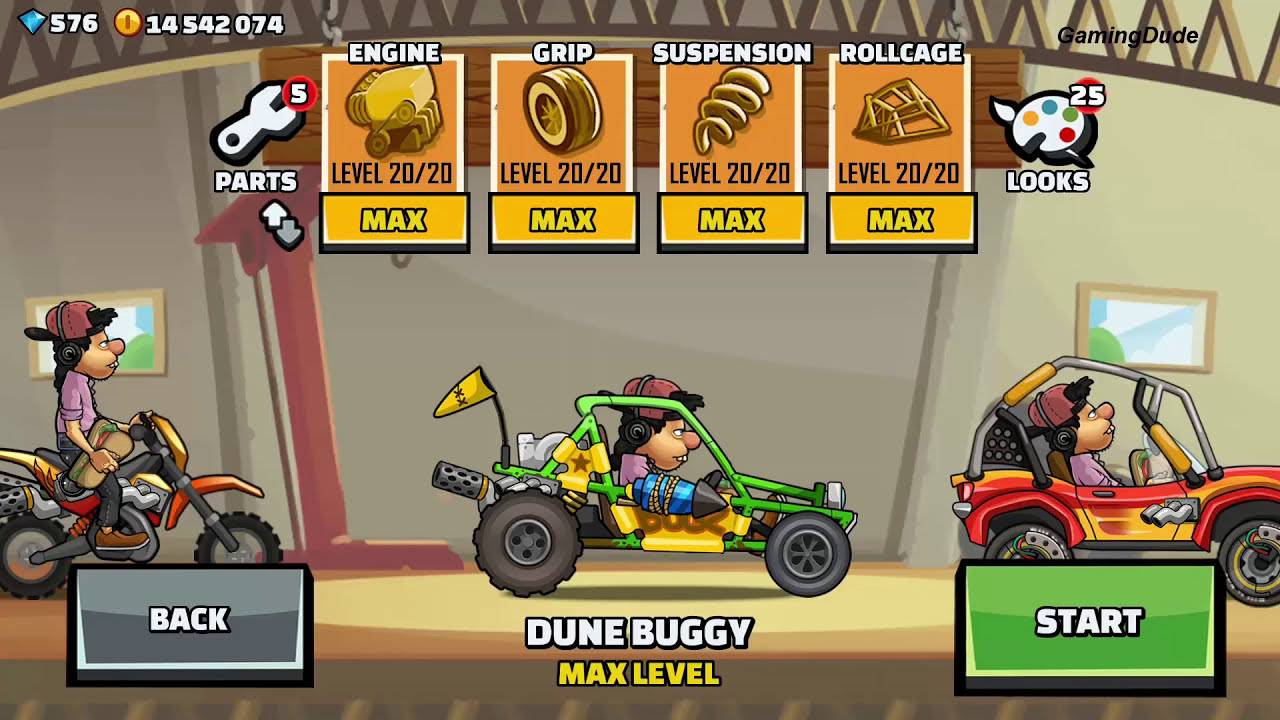This is a detailed screenshot of the opening screen in a game called "Dune Buggy Max Level". The image is a horizontal rectangle featuring various key elements:

At the very bottom, prominently in the center, it displays "DUNE BUGGY" in bold white letters with a black outline. Just below that, in yellow letters with a black outline, it says "MAX LEVEL". Flanking this text, the left side features a black rectangle labeled "BACK" and the right side shows a highlighted green rectangle labeled "START".

The central part of the screen showcases three different cartoon-style vehicles, including a motorbike, and two types of all-terrain vehicles (ATV). Each vehicle has a driver with distinct appearances. The leftmost driver on the motorbike sports a backwards baseball cap and has long hair. The central vehicle, a green dune buggy with a yellow triangular flag, has a driver in a similar style hat. To the right is another ATV with orange, red, and possibly gold hues, and a driver matching the previous two in headgear.

Above the vehicles are four vertical rectangular sections in orange, each corresponding to different parts of the vehicle that have achieved "LEVEL 20-20". These sections are labeled "ENGINE", "GRIP", "SUSPENSION", and "ROLL CAGE", each accompanied by a relevant icon.

On the top left corner, a blue circle displaying the number "576" possibly indicates diamonds, a form of in-game currency. Immediately following is an orange circle displaying "145520174", which might represent a timer or another game stat. Enigmatically inscribed on the upper lattice-like arch is "GAMING DUDE".

To the right side of these sections is an artist's palette with the colors orange, blue, green, and red, labeled with "25". Below this, appears the word "LOOKS".

In the background, the overall color scheme is a muted brown, fitting the game’s theme of off-road adventures and possibly desert landscapes, adding to the immersive gaming experience awaiting the players.